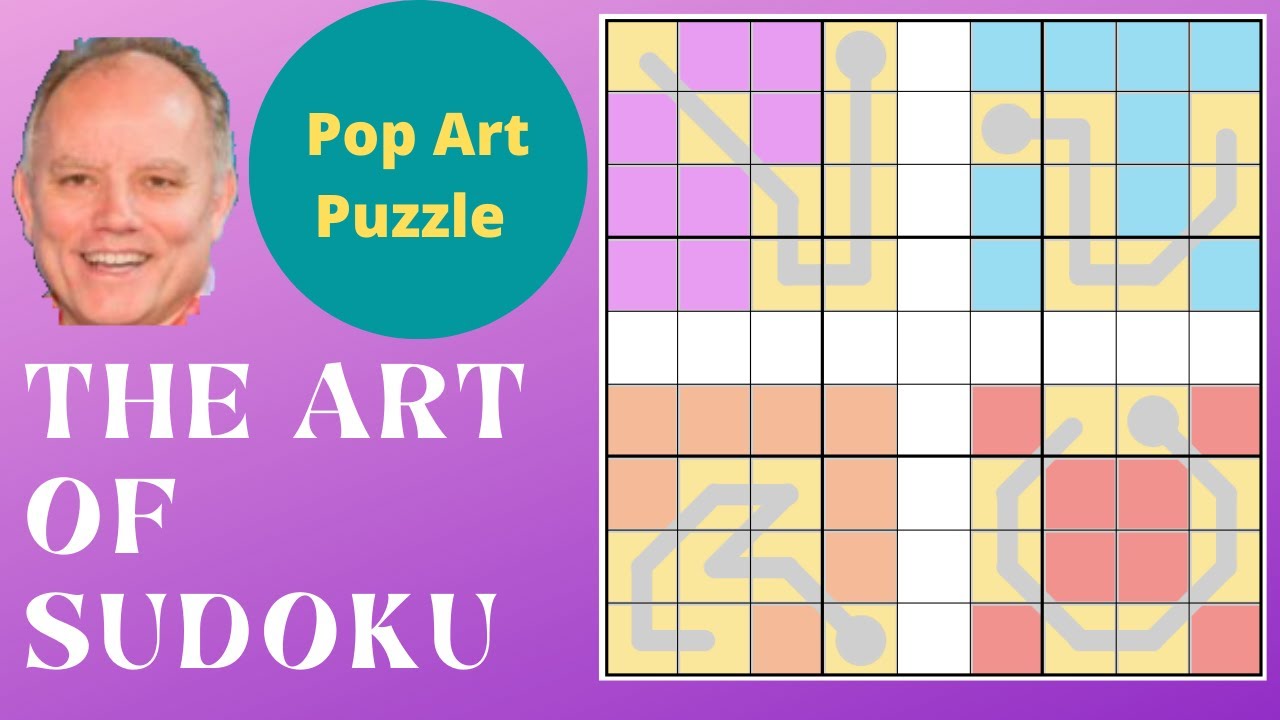The image features a vibrant and detailed cover design for a Sudoku puzzle book. In the top left corner, there's an edited photograph of a Caucasian man with a receding hairline, brown hair on top, and gray hair on the sides near his ears. He has a goofy smile, showing his teeth. Next to his face, towards the right, is a turquoise circle featuring the yellow text, "Pop Art Puzzle." Below this circle, the white text reads, "The Art of Sudoku." The entire background of the cover is a light violet color. On the right side of the cover is a large grid resembling a Sudoku puzzle, consisting of a 3x3 grid pattern made up of smaller 3x3 grids. Several sections of the grid are highlighted in different colors: one is purple and yellow, the adjacent section is light blue and yellow, another is red and yellow, and to the left of that, there's an orange and yellow section. Additionally, there are four gray line patterns creating squares within the grid, adding to the dynamic and colorful design of the puzzle book cover.